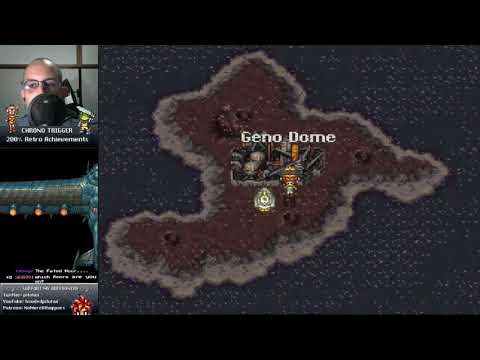This image captures a screenshot of a video game interface, possibly from a Super Nintendo or PlayStation 1 era game, being live-streamed. Dominating the left side of the screen, the top left corner features a small webcam feed of a white, bald, glasses-wearing man speaking into a large microphone against a white background with brown lines. Below this webcam feed, there is a chat bar where viewers are interacting and reacting to the stream. The main part of the screen on the right side showcases a detailed map of a brown island with a lighter brown edge, identifying the in-game location as "Gino Dume." Centered within the map, a character is visible, suggesting active gameplay within the "Chrono Trigger" game. Colors present in the image include black, gray, white, various shades of brown, red, yellow, orange, and blue. The layout indicates a live streaming setup with the webcam in the upper left and the game map occupying the majority of the screen.